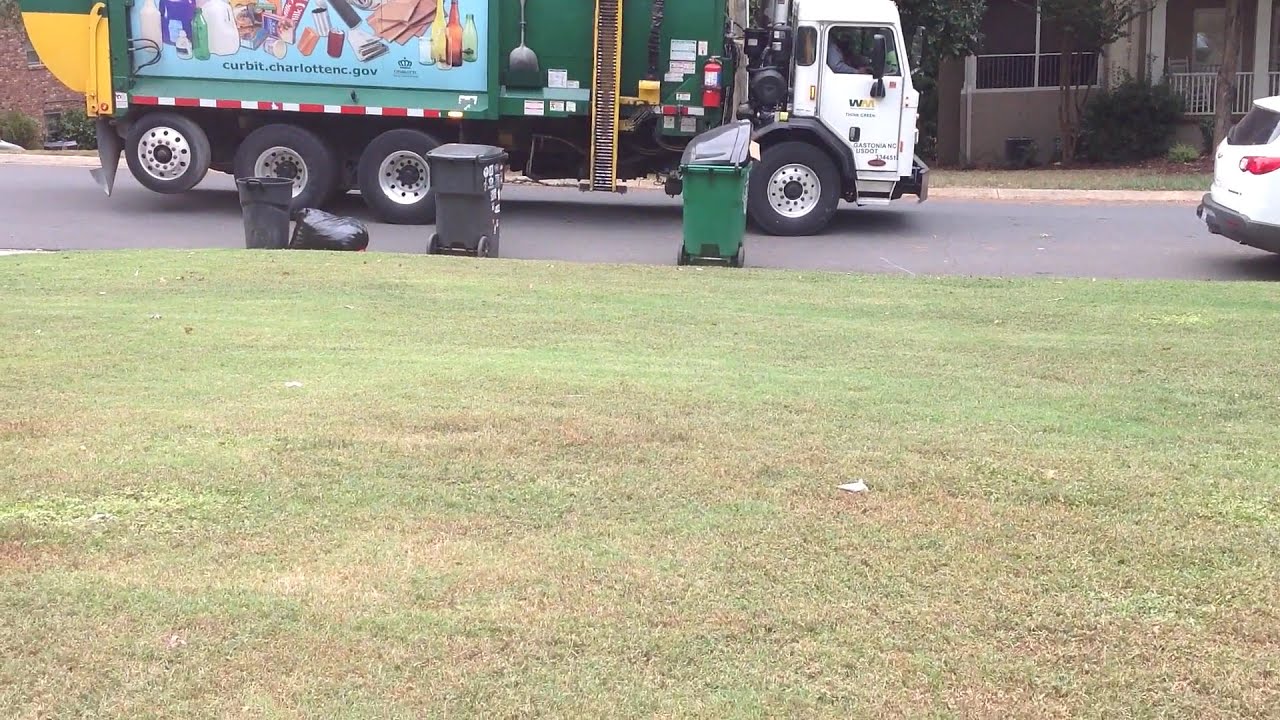In the foreground of this photograph, a large lawn occupies about three-fourths of the image, featuring patches of light green and brown grass. Some white debris—likely pieces of paper or leaves—are scattered on the grass. At the far side of the lawn, lined up along the street, are four garbage bins: three black and one green, the latter possibly designated for recycling. A black trash bag sits beside one of these bins, indicating it remains uncollected.

The upper third of the image displays a garbage truck, characterized by its white cab and predominantly green body with hints of orange or yellow. On the side of the truck is a detailed mural depicting various recyclables, accompanied by the text "curbit.charlottenc.gov" and a waste management logo. Positioned further up the street, the garbage truck is flanked by a white vehicle, potentially a car or crossover.

In the backdrop, beyond the truck, lies a row of single-story houses, one of which features a white porch with a small gate and a door behind it. The image captures a moment seemingly taken from someone's front yard, offering a slice-of-life glimpse into a typical neighborhood scene.